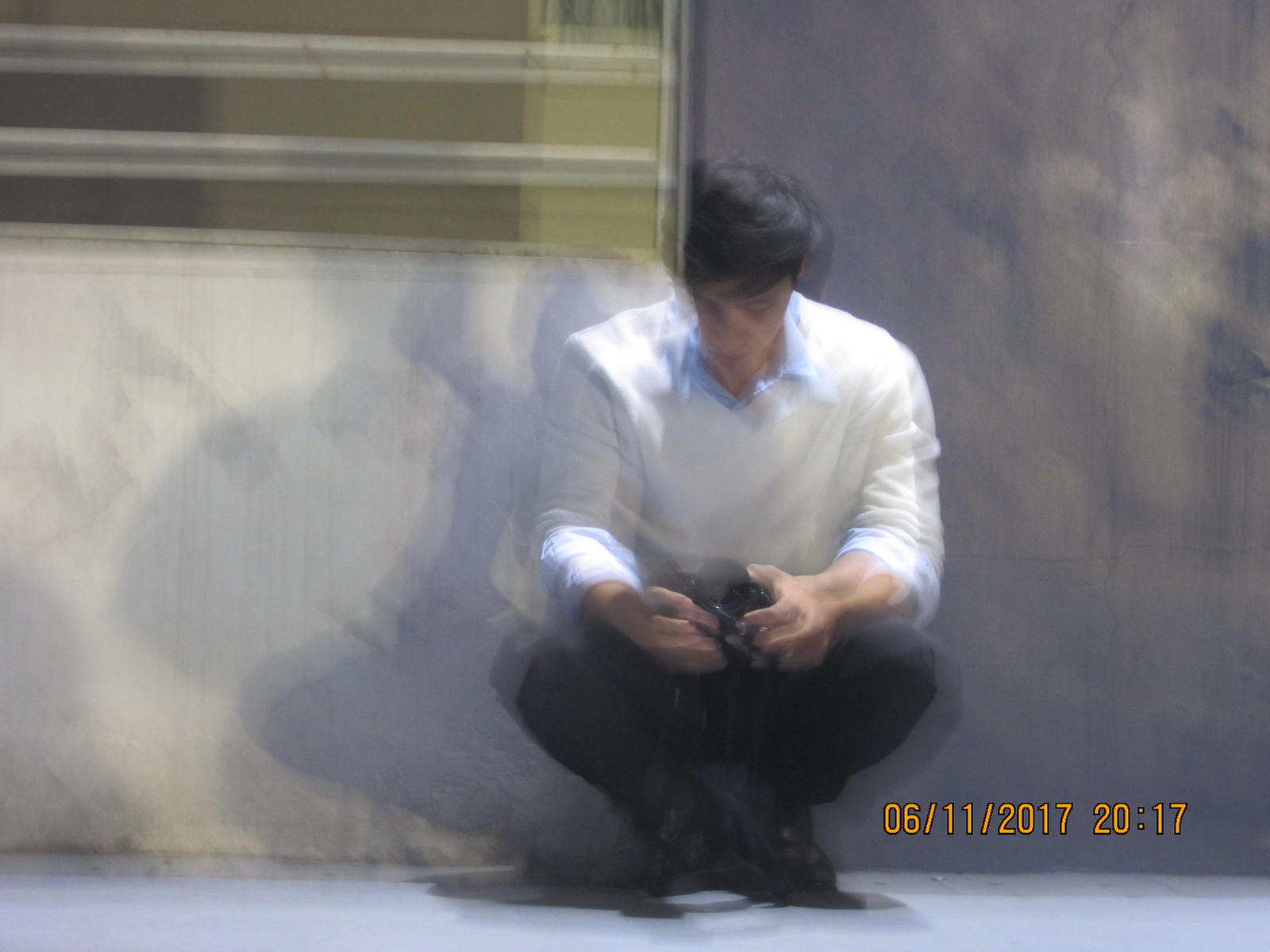In this blurry photograph, a man is captured crouching on a gray sidewalk, likely a street or urban setting. Behind him stands a wall, with the right side appearing dark gray. To the left of the man's head, the wall features a white section that transitions into a yellow, green, and gray area with two vertical white and gray stripes, possibly indicating a window. The man is attired in black pants, black shoes, and a white shirt with a noticeable blue collar. His dark brown hair suggests he might be young or middle-aged. He appears engrossed in an object he holds in his hands, seemingly in motion. The date "06-11-2017" is visible, presumably marking when the picture was taken.